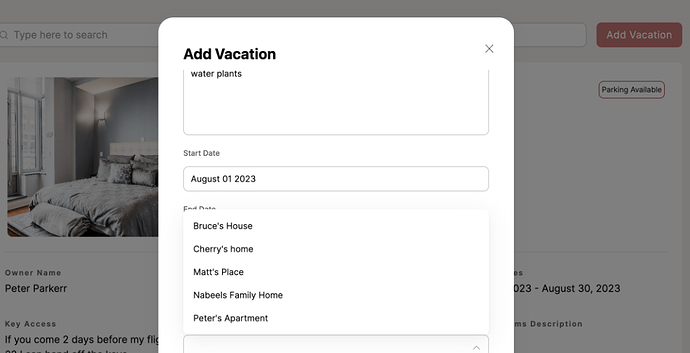**Caption:**

In the center of the image, a window is prominently featured, hinting at a vacation destination with water plants visible outside. The top right corner of the image contains the text "X" and "Start Date: August 1st, 2023." The visual includes depictions of several residences, specifically Bruce's house, Cherry's home, Matt's place, Nabila's family home, and Peter's apartment.

The top left corner displays a bar, and adjacent to it in the top right center area, the word "Advocation" is shown. On the left side, there is a note indicating "Parking Available." In the bottom left, another window is depicted, through which a bed with gray sheets and pillows can be seen.

At the bottom of the image, under the name "Peter Parker," it is mentioned that key access will be available if arriving two days before the start date. The bottom right corner displays "23-2, August 30th, 2023." Finally, the left side also includes a section labeled "Description," and a gray filter overlays the entire image, adding to its subdued tone.